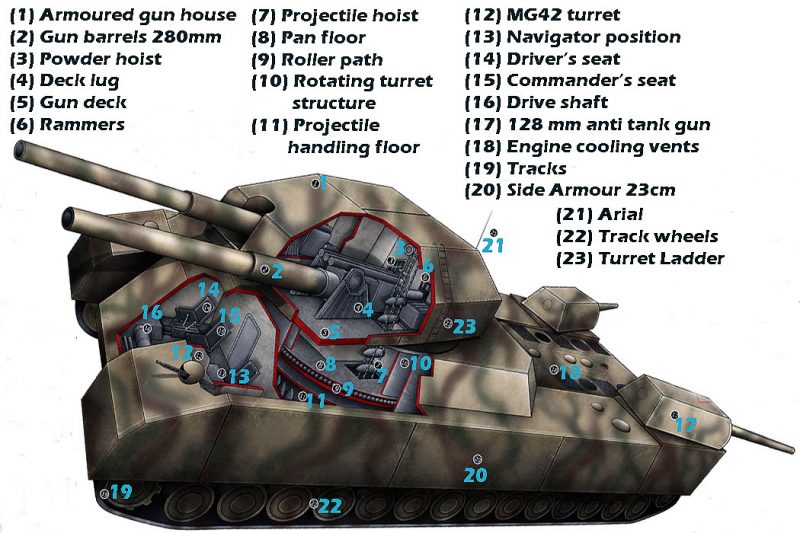The image is an animated and detailed breakdown of a tank design, similar to a video game or toy model. The tank, depicted in a grayish-black color, features a large turret on top with two prominent cannons pointing left. Additionally, there are two smaller turrets on the back end aiming right. The tank moves on a tread system visible from above, though the underside is not shown. The illustration includes transparent sections to reveal interior details, such as seating arrangements and arsenal placements. The tank is adorned with 23 numbered characteristics, highlighted with light blue numbers on the tank itself and detailed in corresponding black font above the image. The view is an elevated front-left angle, providing a comprehensive look at both the exterior and key internal components, ensuring a thorough understanding of the tank's features and layout.